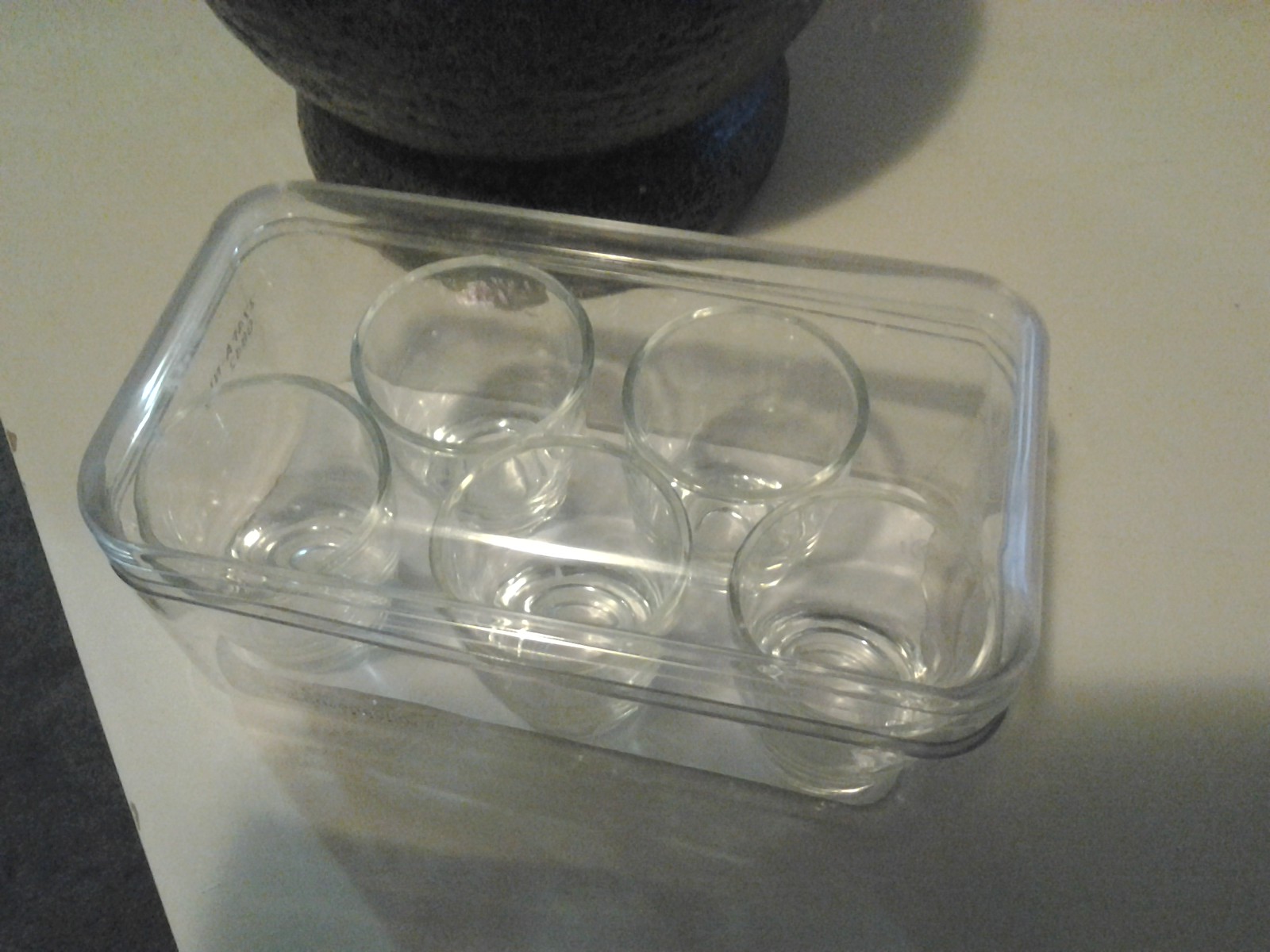The image features a transparent, glass container with a rectangular, rounded-edge design, positioned on a white countertop. Inside the container are five small drinking glasses, likely shot glasses, arranged with two in a top row and three in a bottom row. The container appears to have a lid, although the text on the left side of the container is too small to discern. In the background, there is a large, black cylindrical object with a round, spherical shape and a medium-sized base, mostly out of frame, resembling the base of a stone bowl or possibly the bottom of a mortar and pestle. Additionally, two small chips can be seen in the darker part of the lower left section of the countertop, with something black on the floor in the same area.